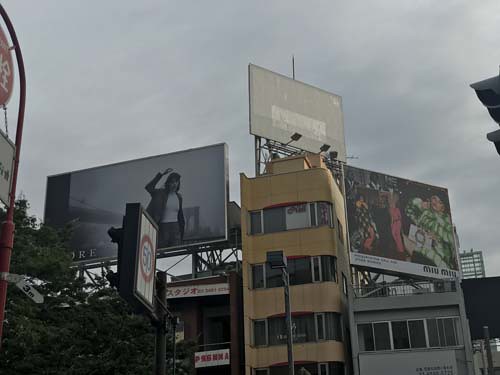In this photograph of an urban cityscape, several billboards top the buildings, each advertising different messages. One prominent billboard features an individual in a jacket raising their arm against a foggy backdrop, though the product or service being promoted is unclear. Another conspicuous sign displays the number "50" encircled in red, likely indicating a route number for a nearby road. 

Amidst the hustle and bustle, a tan building stands ahead, juxtaposed against a street light that illuminates the scene. Another billboard advertises a company, potentially named "MIU," showing people gathered in a room. An additional sign, written in Asian characters with a red text on a white background, adds to the cultural diversity of the environment. Above, a cloudy overcast sky looms over the urban landscape, setting a contemplative mood over the bustling city below.